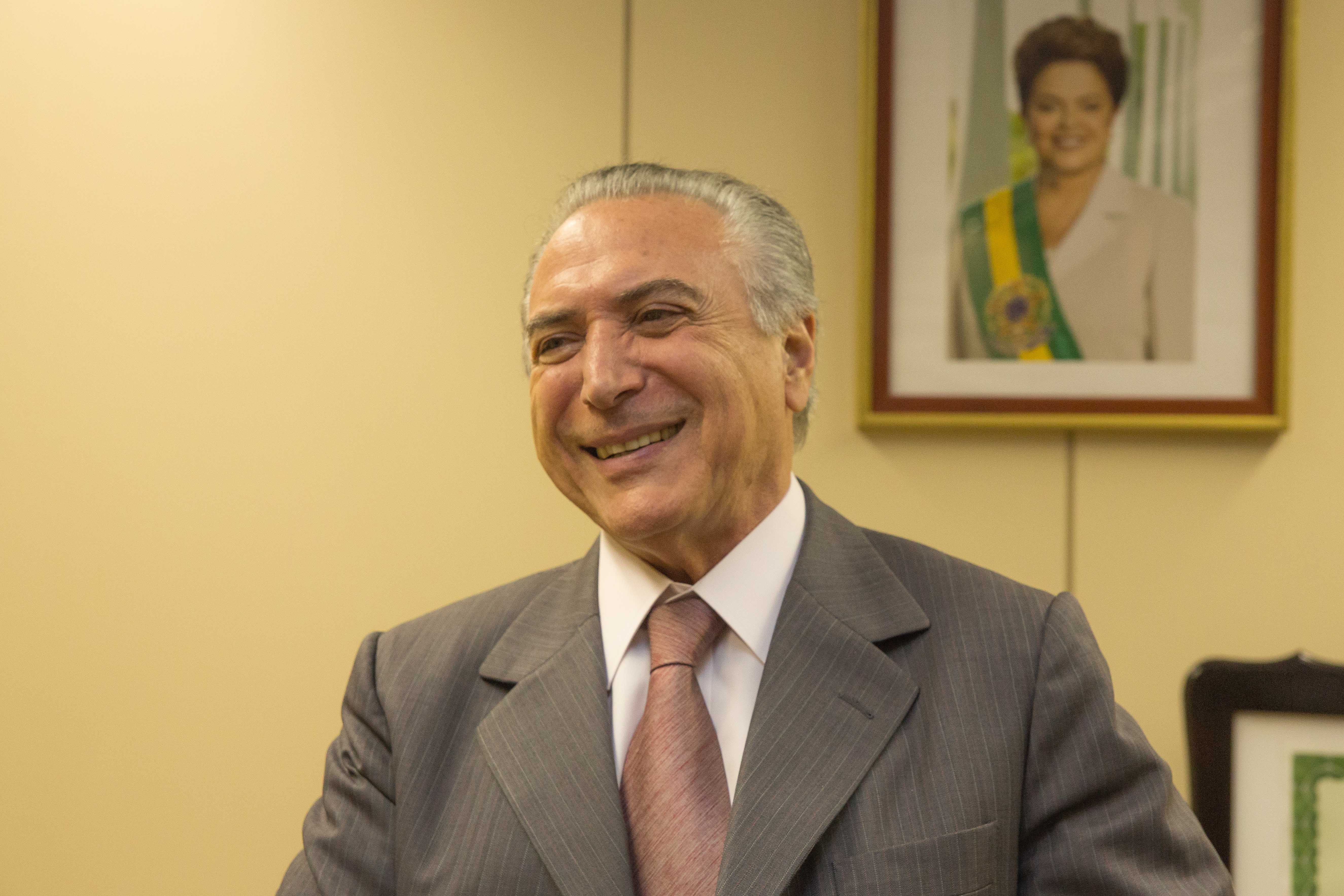The photograph features a professional-looking man, possibly a politician, with neatly groomed gray hair and gray-brown eyebrows, slicked back stylishly. He is dressed in a subtly striped dark gray suit paired with a collared white dress shirt and a faded red tie. His expression is a broad smile, revealing pursed lips and teeth, and he is gazing off towards the left distance rather than directly into the camera. The man exudes a composed demeanor with a few wrinkles around his eyes, adding character to his appearance.

In the background, a stately woman is prominently featured in a framed photograph. She has poofy dark hair and is adorned in a long-sleeved white dress, accentuated by a professional-looking ribbon or sash draped over her shoulder, which might signify some official status or honor. The room has light yellow or perhaps cream-colored walls, influenced by the lighting, with subtle lines that add texture to the setting. There is also another painting situated lower on the wall, adding to the scene's complexity and richness.